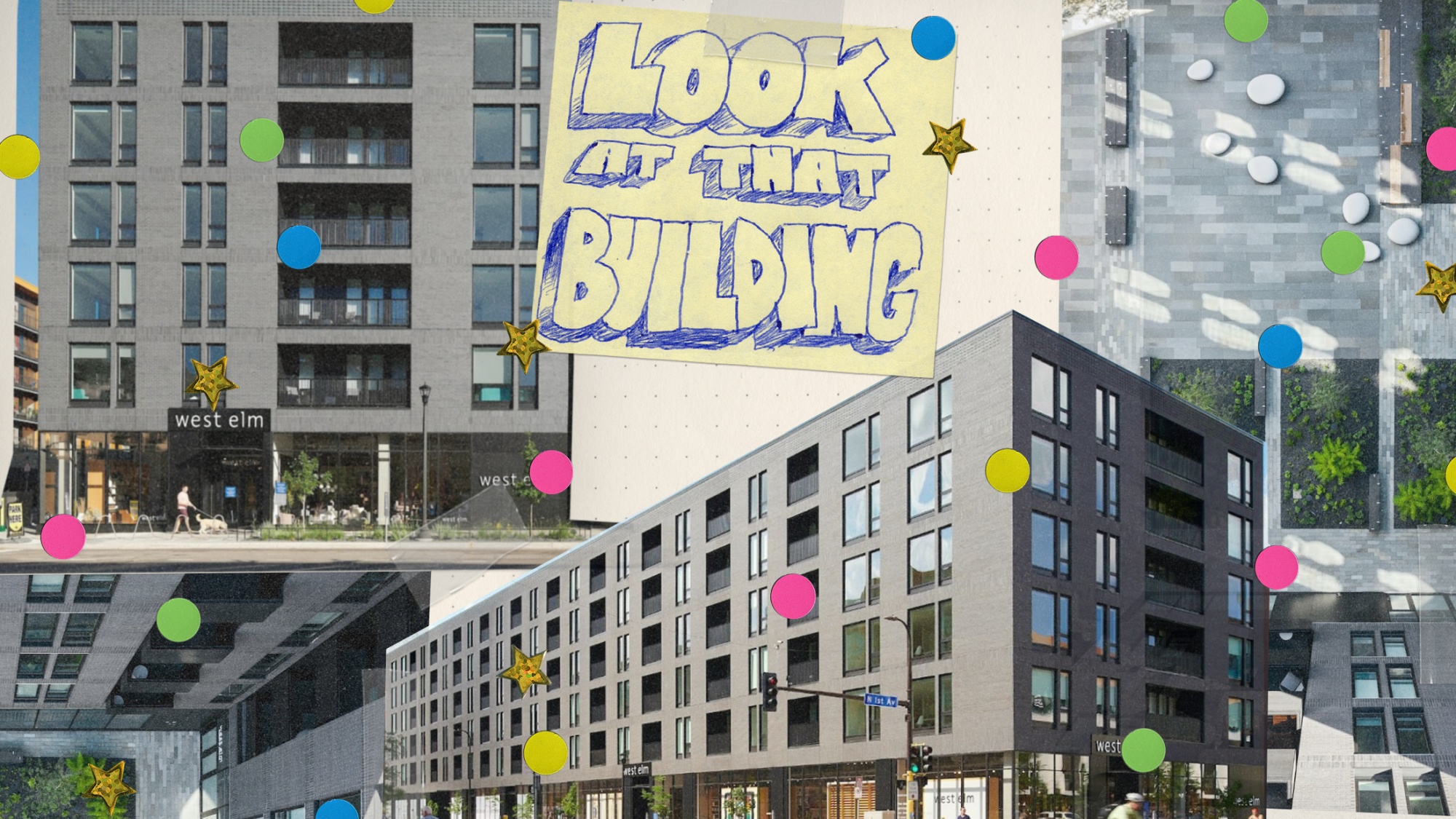This is a detailed artist's sketch collage featuring multiple gray, square, multi-story buildings, approximately five stories tall, not including the ground floor. The buildings are illustrated with various textures, including a brick texture in the building on the upper right. Overlaid on the collage are numerous colorful dots and stars in blue, pink, yellow, and green, seemingly marking points of interest. 

In the top left corner, there is a building labeled "West Elm" above its front doors. This building showcases balconies on each floor and windows flanking the balconies. The top center of the collage features a sticky note with cartoonish bubble letters that read "Look at that building." 

The bottom left displays a bird's eye view of an inner corner of a building, highlighting a green area with a walkway and floral arrangements. A green dot marks one of the balconies. The bottom center presents a full-length view of another building, emphasizing clear, large windows on the ground floor, alongside scattered dots marking specific areas. 

A man is seen walking on the street, and there's a dog nearby, adding life to the scene. The upper right also offers a close-up of a similar building with colored dots and white ovals indicating marked features. Green shrubbery and bushes are visible near the building's ground. Overall, the collage combines views from different angles, enhancing its intricate and detailed nature.